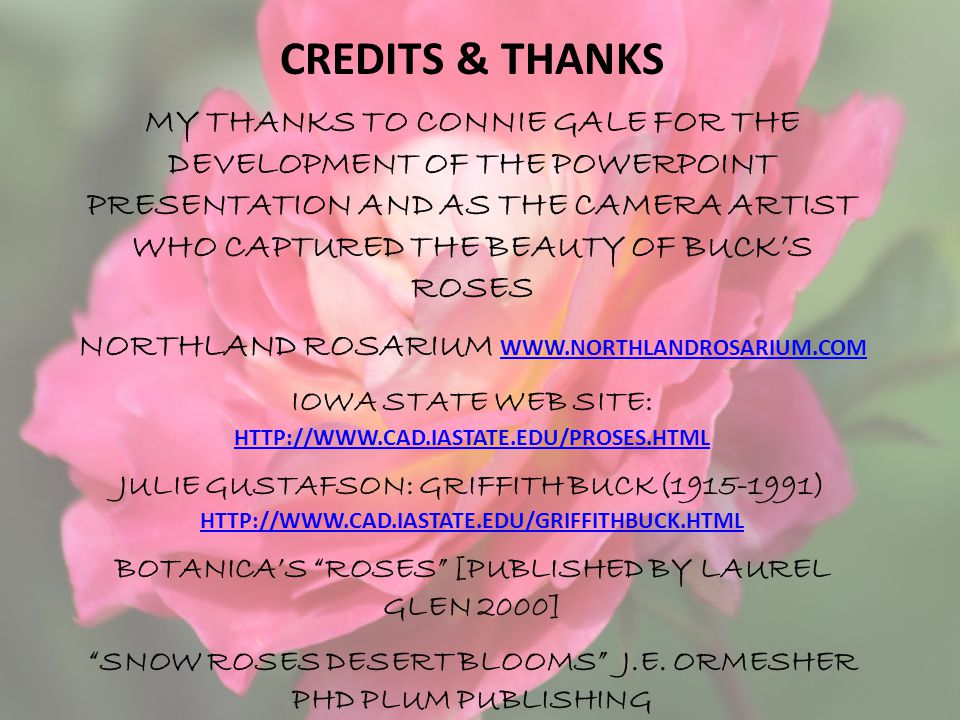The image features a vibrant pink flower with a white center, set against a blurred green background that includes leaves and a stem. The flower dominates the photo, centrally positioned, and the photo serves as a PowerPoint slide with text overlaid. At the top of the slide, in all capital letters, it says "CREDITS AND THANKS," where "AND" is represented by an ampersand. Below this header, the slide expresses gratitude to Connie and Gail for developing the PowerPoint presentation and for serving as the camera artists who captured the beauty of Buck's roses. Following this acknowledgment, various sources and contributors are listed, including "Northland Rosarium" (www.northlandrosarium.com), the "Iowa State website" with a specific URL, and "Julie Gustafson Griffith Buck (1915-1991)" with another URL. Additionally, it cites "Botanica's Roses, published by Laurel Glen in 2000," and "Snow Roses, Desert Blooms by J.E. Ormesher, Ph.D., published by Plum Publishing." The text is centered and alternates between black and blue, with some portions underlined, filling the entire image while emphasizing the written content.